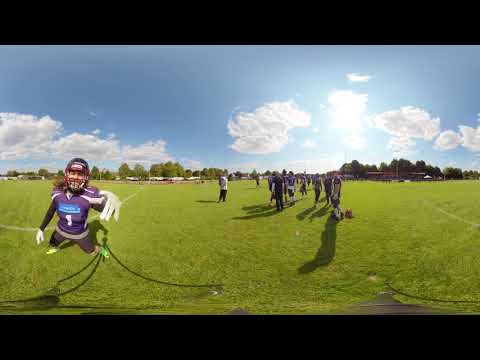This horizontal rectangular image features a dynamic outdoor scene, framed by dark borders at the top and bottom. The foreground is dominated by a vibrant, healthy green field of grass, while the upper half of the image showcases a striking blue sky adorned with large, white, fluffy clouds. A bright sun illuminates the scene from above, casting light over the entire landscape.

On the left side of the image, a figure draws attention. This individual, dressed in what seems to be lacrosse equipment, is prominently positioned close to the viewer, appearing to float above the ground, suspended by an unseen attachment. The person is clad in purple attire, complete with a number on their shirt and a white towel draped over their arm. The enigmatic nature of the figure's position suggests an unusual activity, possibly capturing a drone selfie.

To the right, several smaller figures stand on the field, observing the scene. Although they are not clearly discernible, their presence adds to the image's sense of curiosity and wonder. The horizon is lined with a scattering of trees, enhancing the natural beauty of this vibrant and surreal outdoor setting.